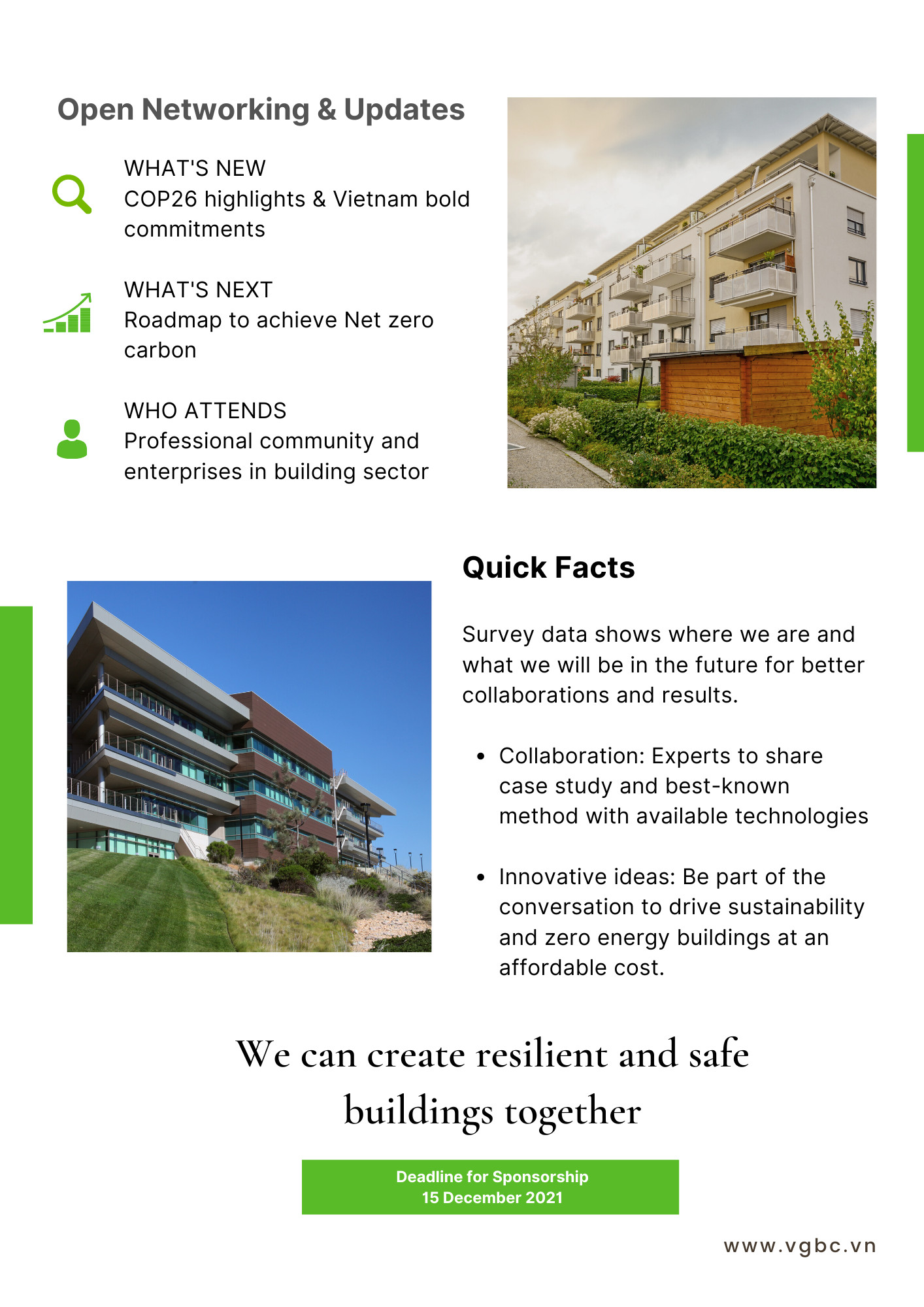This vertical rectangular image is an informational poster detailing updates and initiatives for COP26, with a particular focus on Vietnam. At the top of the image, the title is displayed in black text: "Open Network and Updates." Below this headline, in all capital letters, are the words "WHAT'S NEW?" followed by "COP26 HIGHLIGHTS," and "VIETNAM: BOLD COMMITMENTS." A green magnifying glass icon is situated to the left of this section.

The next section, beginning with "WHAT'S NEXT?" in all capital letters, outlines a "roadmap to achieve net zero carbon," featuring a green icon resembling a bar graph with an upward arrow on the right.

Following this, "WHO ATTENDS" is stated in capital letters, highlighting the "professional community and enterprises in the building sector." To the left of this text is a green icon depicting a person. Adjacent to this section is a vertical image of an apartment building.

A thick green vertical line divides this portion from another segment on the left side of the image, which includes a thicker vertical green line to the left of another image of apartment buildings. This second image is characterized by a bright blue sky and a green lawn.

To the right of these images, "QUICK FACTS" is written in bold black font, followed by a detailed description in regular black font: "Survey data shows where we are and what we will be in the future for better collaborations and results." The section lists key points in bullet form:
- *Collaboration*: "Experts to share case study and best known method with available technologies."
- *Innovative Ideas*: "Be part of the conversation to drive sustainability and zero energy buildings at an affordable cost."

Centered at the bottom of the image is a motivational statement in larger, bold black font: "We can create resilient and safe buildings together." Beneath this, in a horizontal green rectangle with white lettering, the text reads: "Deadline for Sponsorship: 15 December 2021." Lastly, in smaller black font towards the bottom right, the website URL is listed: "www.vgbc.vn."